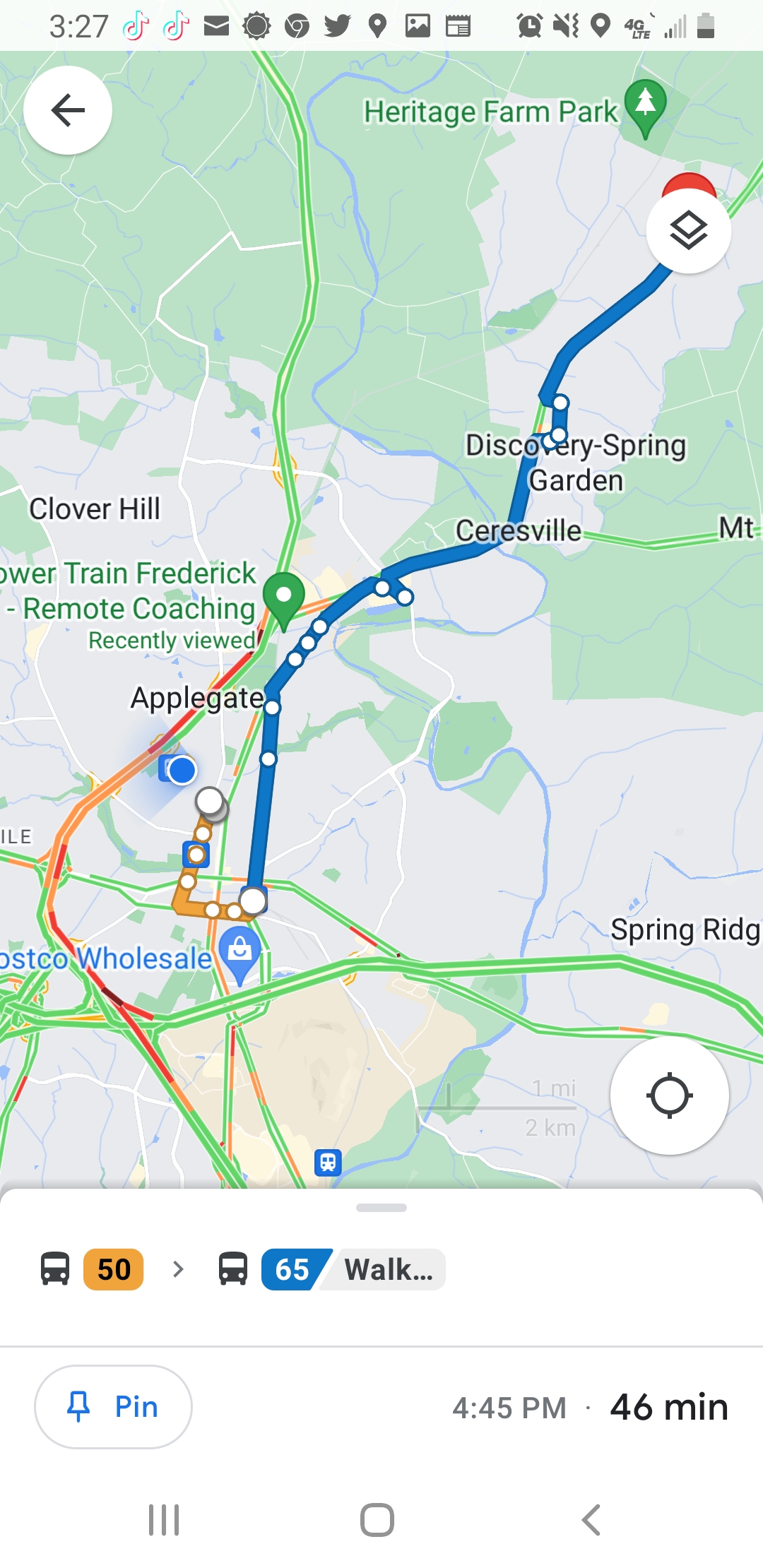This detailed screenshot of a mobile device, likely an iPhone, displays a vibrant, color-coded map from a mapping app. The map outlines a route marked by a prominent blue path, indicating a potential bus route or pedestrian walkway. At the top left corner, the device's status bar shows the time as 3:27 PM and various app icons, suggesting additional functions available on the device.

The mapped route starts at Heritage Farm Park, identified by a green pin suggesting a National Park. Traveling down, the route passes through Sarasville and Discovery Spring Garden. Applegate is also noted along this blue path, possibly indicating another point of interest or stop. To the left, an arrow points towards a remote coaching facility, with 'Clover Hill' labeled above it. 

Near the bottom of the map, two green-highlighted roadways are visible, leading to Costco Wholesale and Spring Ridge. Additionally, a small white tab at the bottom holds a bus icon with '50' in a yellow bubble and '65' in a blue bubble, indicative of bus numbers. Adjacent to this are the words 'Walk...' suggesting an alternative route or option. 

Further below, the tab displays the time (4:45 PM), and an estimated travel duration (46 minutes). At the very bottom, the typical mobile controls—a backwards arrow, home button, and a multitasking icon—are visible, confirming the mobile nature of the device. This cohesive layout serves to guide the user through various waypoints and destinations with precision and clarity.